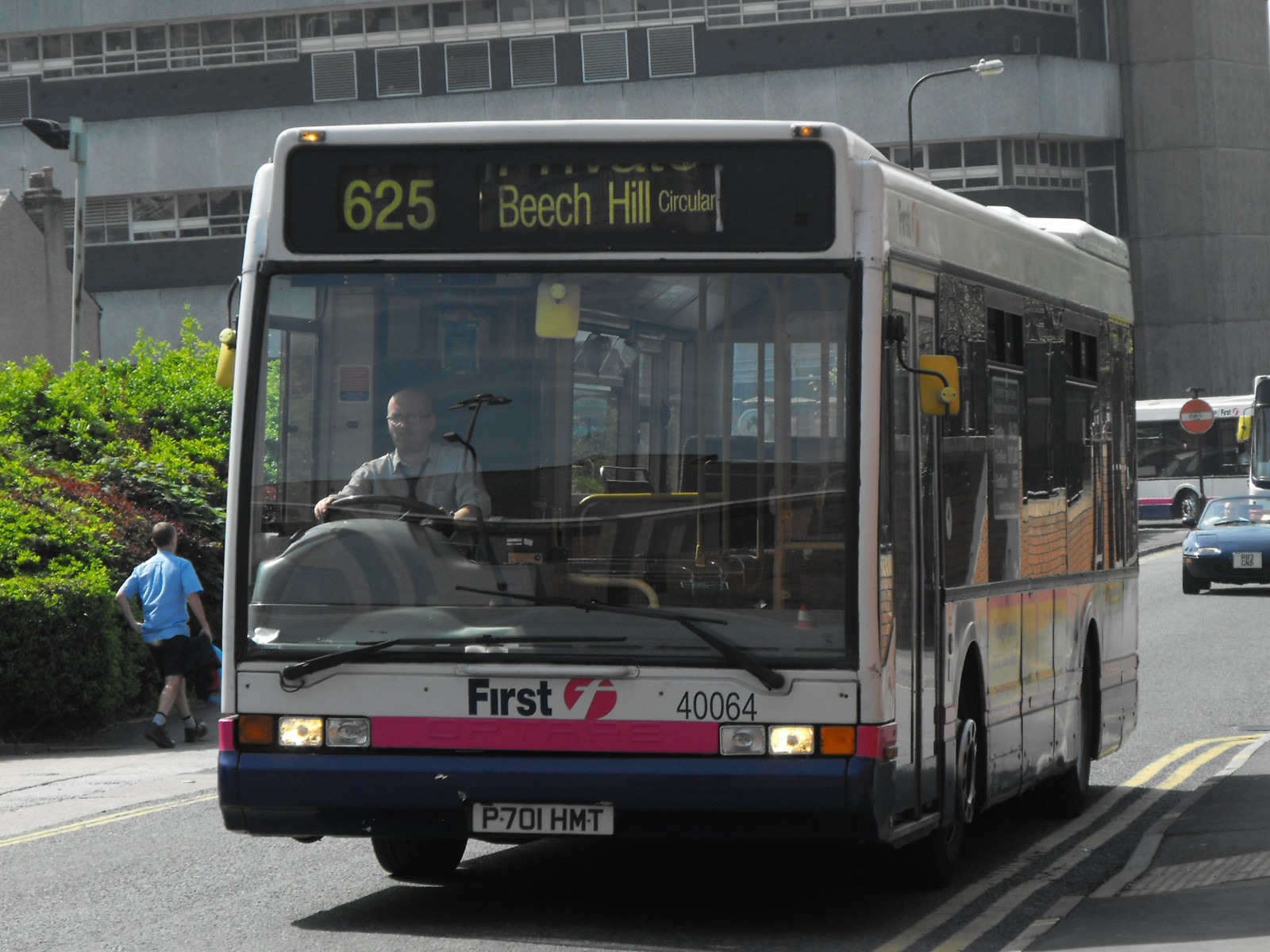The image captures a city bus traveling toward the camera on a street that is not very busy. The white bus, prominently displaying the route number 625 to its destination, "Beach Hill Circular," is equipped with large front windows and electronic signage above the windshield. The driver, visible through the windshield, is wearing a light button-down shirt with a loosened dark necktie and has both hands on the wheel. The bus is empty, with no passengers visible inside.

The bus features the logo "FIRST" in black letters beneath the windshield, indicating the transit authority, along with a small, pink T-shaped symbol. The vehicle bears the license plate number P701 HMT, resembling a European-style plate. The headlights are turned on, illuminating the street ahead. To the left of the bus in the image, there's a pedestrian dressed in a blue t-shirt and dark shorts walking past a line of bushes. Behind the bus is a red convertible, possibly a Miata, and in the background, there is a large building with windows and a wall of hedges or green grass. The photo provides a detailed snapshot of the bus's journey and its surroundings.